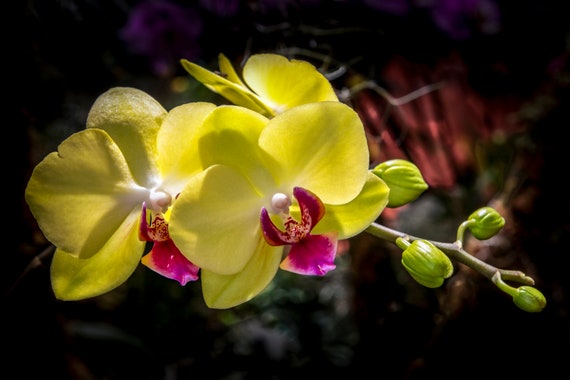This detailed nighttime macro photograph captures the striking beauty of a yellow orchid in full bloom. The flower, which serves as the focal point, features six vivid yellow petals and a unique pink "lady slipper" center adorned with delicate white dots, giving the impression of a pearl nestled within. Surrounding this main bloom, there are additional blossoms—three or four fully open and at least four or five still in the bud stage, yet to unfurl. These unopened buds are a vibrant green, contrasting with the mature flowers. The background is a blurred, almost mystical black with subtle maroon and purplish hues around the edges, enhancing the orchid's radiant colors and making them pop amidst the darkness. The light green stems add a fresh touch to this enchanting image.